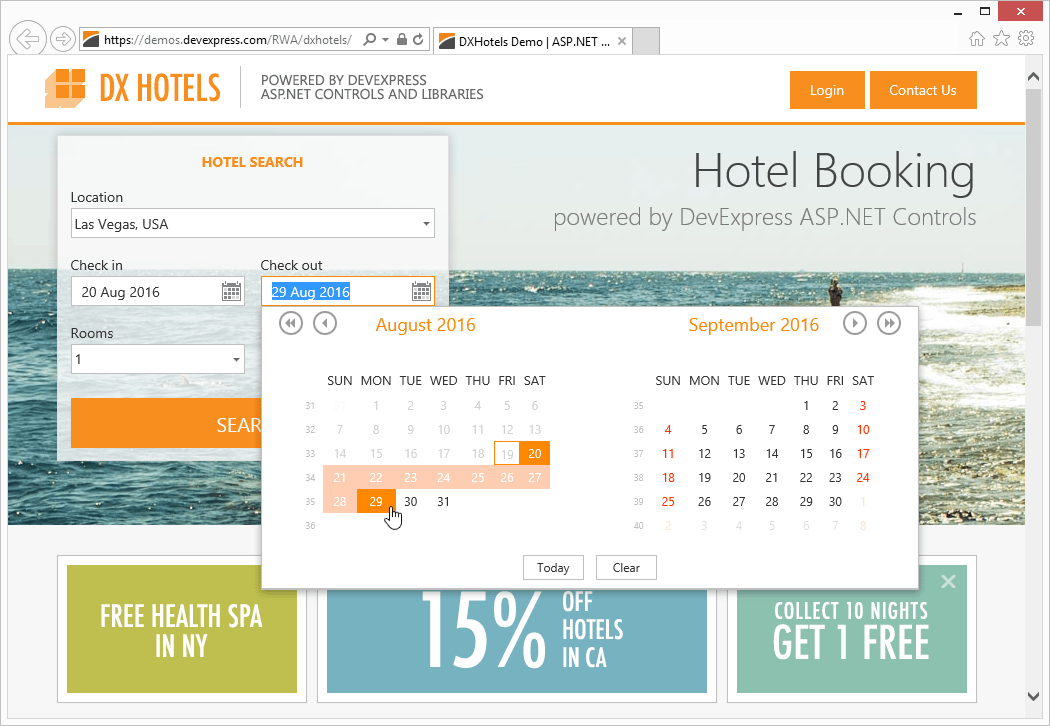Caption: 

Screenshot of the DX Hotels website, showcasing a powerful interface powered by DevExpress ASP.NET controls and libraries. The focused pop-up allows users to select their booking dates with selections for August and September 2016, featuring buttons labeled "Today" and "Clear". Behind the pop-up, the primary interface displays a hotel search form with details including location set to Las Vegas, USA, check-in date of August 20th, and check-out date of August 29th. A picturesque image of someone walking along a beach is subtly visible in the background, creating a serene aesthetic. Beneath the main interface, there are promotional links for additional offers: "Free Health Spa in New York," "15% Off Hotels in California," and "Collect 10 Nights, Get One Free."